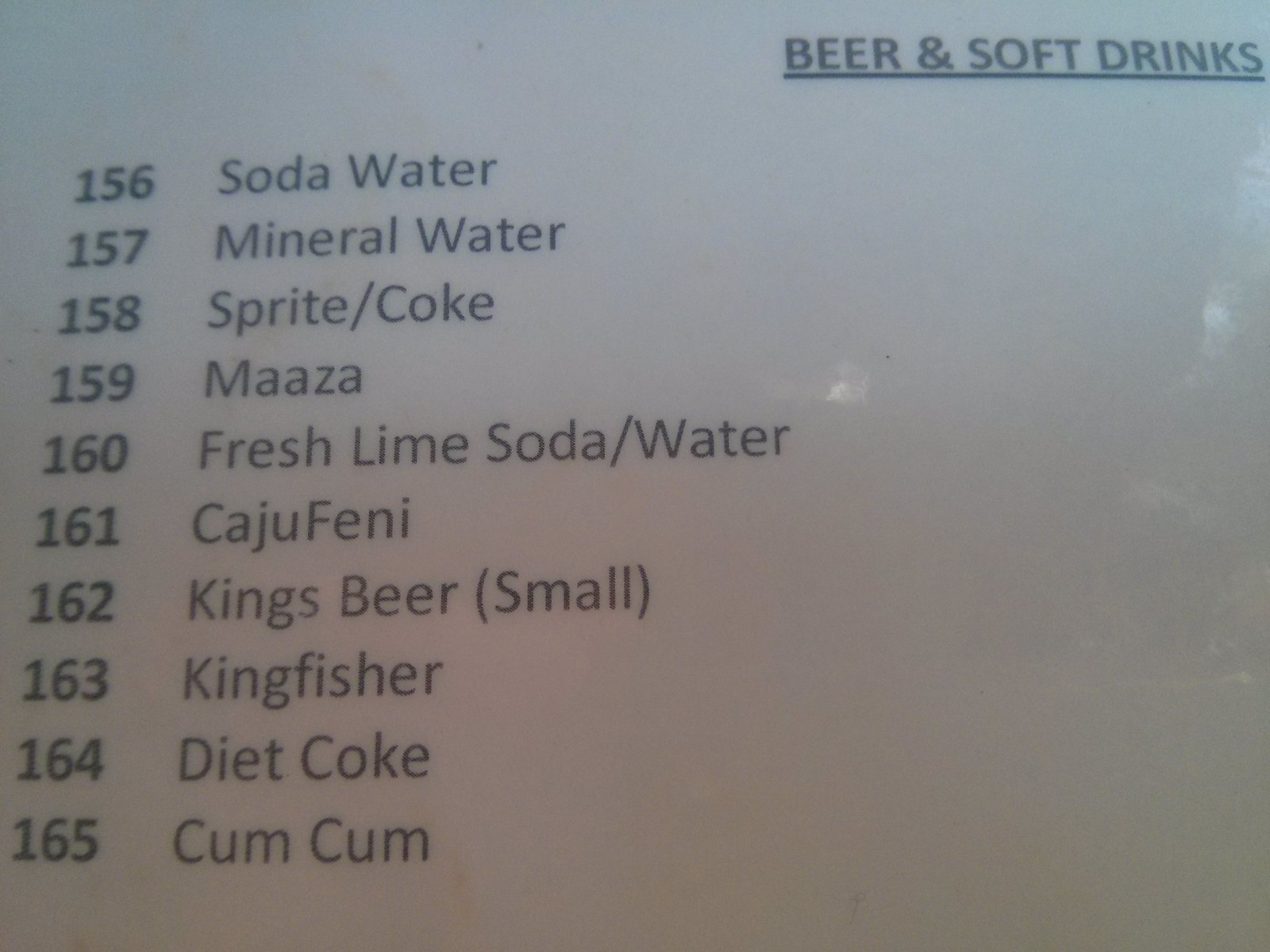The image depicts a menu-like piece of paper with a white background and black text. At the top, in bold, all-caps, and underlined, it reads "BEER AND SOFT DRINKS." Below this heading, the list begins with the number 156 in the left column and proceeds sequentially down to 165. Each entry on the left is followed by the name of a drink in the adjacent column. The drinks listed are: 

156. Soda Water,
157. Mineral Water,
158. Sprite/Coke,
159. Mazza (spelled M-A-A-Z-A),
160. Fresh Lime Soda/Water,
161. Caju Feni (spelled C-A-J-U-F-E-N-I),
162. King's Beer (small),
163. King Fisher,
164. Diet Coke,
165. Cume Cume (spelled C-U-M-C-U-M).

The text appears as if typed on a computer.